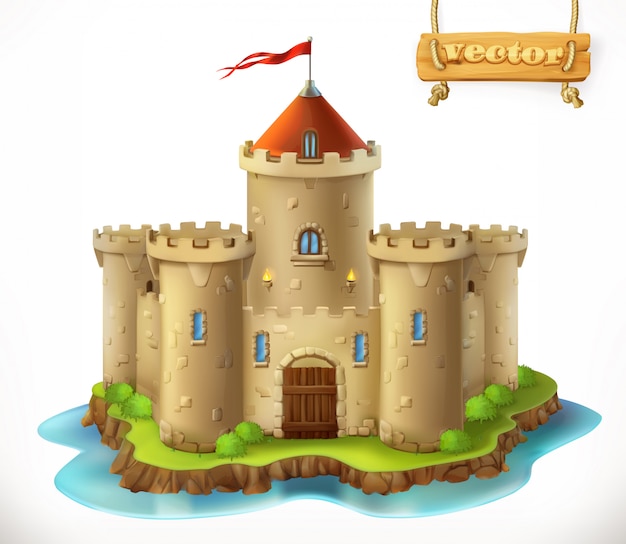The image depicts a detailed 3D render of a cartoonish medieval castle set on a small green island surrounded by a bright blue moat. The castle is primarily gold in color and consists of five towers: four shorter exterior towers and one taller central tower. The central tower, distinguished by a pointed red roof, prominently features a red flag at its apex, two windows, and flanking torches. The castle's structure includes tall stone walls forming a circle around the main tower, with small bushes interspersed along the edges. The foreground showcases a wooden gate, which is actually a raised drawbridge, adding to the fortress-like appearance. In the upper right corner of the image, a wooden sign held by two ropes hangs, clearly displaying the word "vector," adding an additional touch of whimsical detail to the scene. The entire composition evokes the feel of a toy or a playful, animated setting.